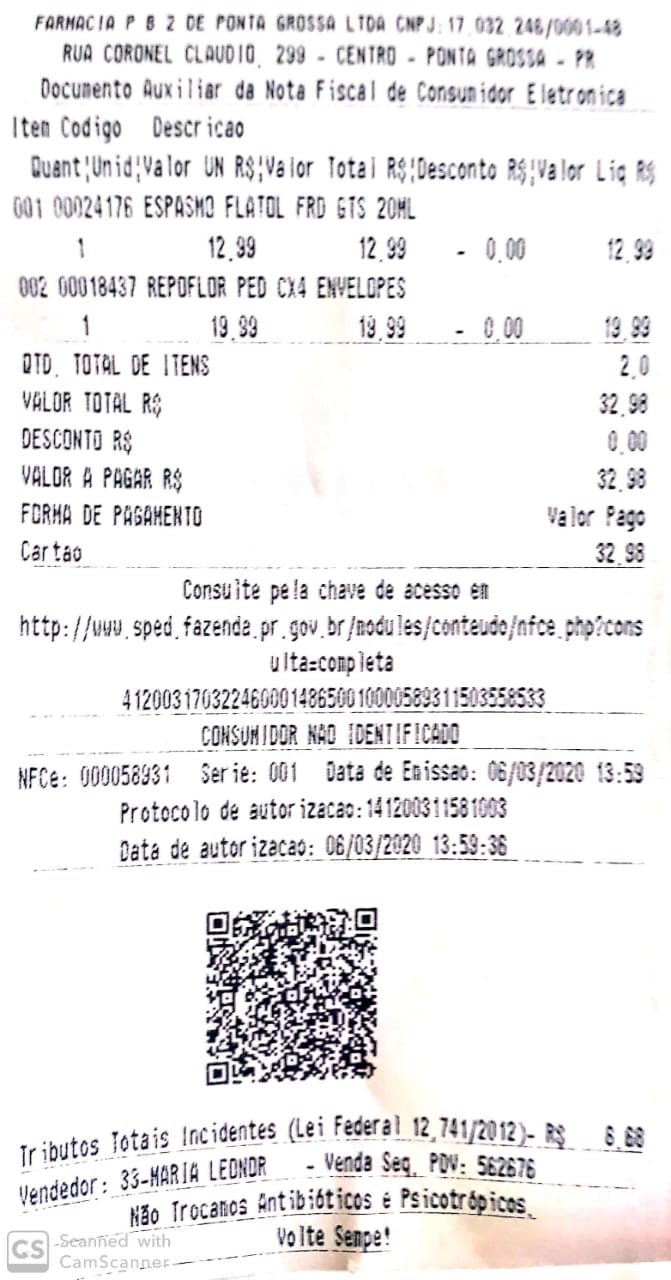A detailed image caption for the described receipt:

"This image showcases a retail receipt, primarily written in Spanish, titled 'Documento Auxiliar de Nota Fiscal de Consumidor Electrónica.' The receipt details two purchased items, one priced at $12.99 and the other at $19.99, making the total for both items $32.98. However, it does not specify the payment method used. The receipt includes miscellaneous details, such as a QR code and an unidentified logo in the bottom left corner. The entire image appears to have been scanned using the CamScanner app, as indicated by the watermark."